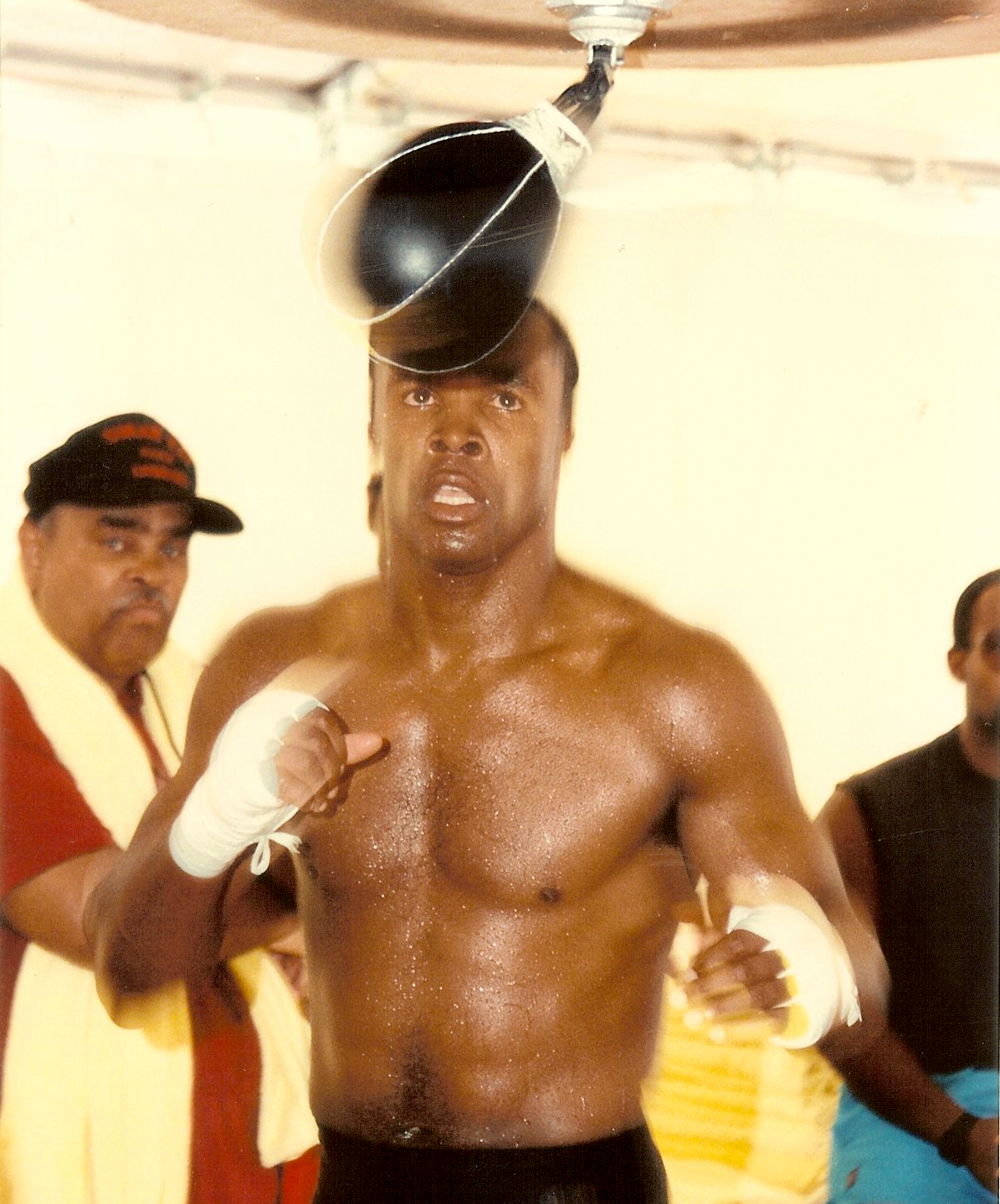This image captures a professional black male boxer shirtless in a gym, caught mid-training as he strikes a small, black punching bag positioned above head height. His hands are meticulously wrapped in bandages, and he is dressed in black shorts. The boxer is surrounded by two men. To the left, a black male trainer with a mustache wears a bright yellowish off-white towel draped around his shoulders and a red t-shirt with a black baseball cap featuring red writing. Another man appears on the right side but is partially cut off; he wears a black sleeveless shirt and blue shorts. The background is a typical boxing gym environment, reflected in the muted, somewhat faded colors of black, white, brown, beige, yellow, red, and blue. Despite the possible paparazzi shot style, the image lacks clarity and focus, giving it a candid, raw appeal. Unreadable text is also present in the background.